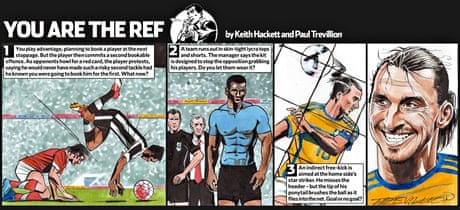This detailed caption merges and highlights the universally mentioned and recurring elements from multiple descriptions:

---

The image is a four-frame comic strip titled "You Are the Ref," created by Keith Hackett and Paul Trevelyan, renowned for blending real-life football scenarios with illustrated storytelling. In the first frame, a dynamic soccer scene portrays a player in a red jersey on the ground and another player in a black and white striped jersey skillfully landing on his hands over a soccer ball. The second frame features three distinct figures— a coach, a referee dressed in black with a white insignia, and an athlete in a blue shirt and shorts, likely a soccer player, participating in what appears to be a referee's decision-making moment. Moving to the third frame, we spotlight another soccer player, wearing a yellow and blue jersey labeled with the number 10, energetically heading a soccer ball through the air, his hair flying to convey motion. The final frame zooms in on this same athlete, now depicted with a broad smile. Notably, this character resembles Zlatan Ibrahimović, adding a touch of real-world recognition to the comic strip's immersive portrayal of soccer dynamics.